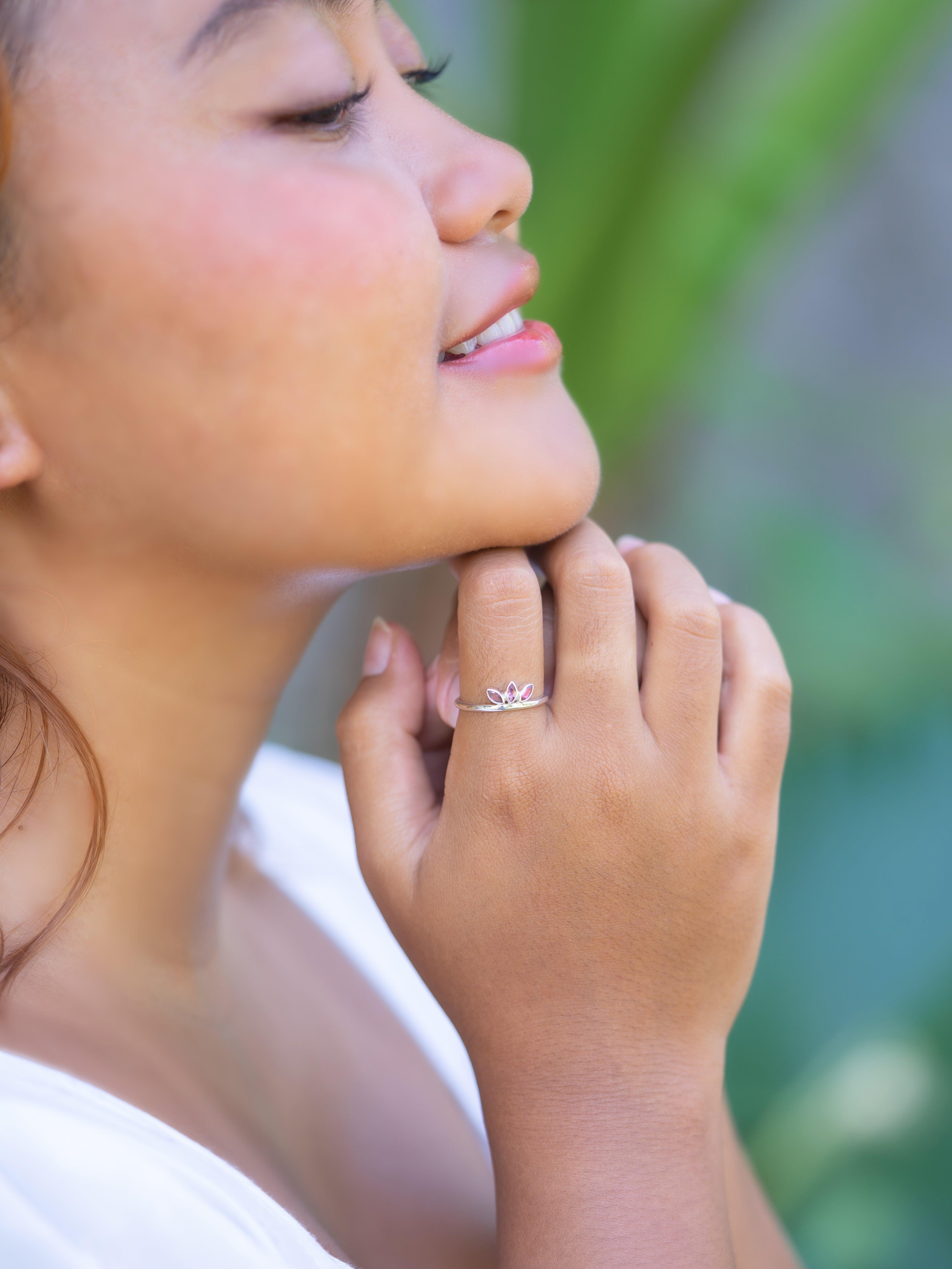This is a color photograph of a young woman with a slight tan and Southeast Asian features, possibly Filipino. She occupies the left side of the portrait-oriented image, which captures her from just below her shoulders to the top of her eyebrows. The background is a blurred, dark green, likely indicating foliage. The woman is facing left and looking downward with a gentle smile, revealing her slightly open mouth and white teeth. Her dark hair has a wisp gently touching the right side of her neck, and her long, brown-black eyelashes frame her barely open eyes. She wears a white scoop-neck top and her hands are clasped just below her chin. On her pointer finger, she wears a silver ring with three floral petals adorned with pinkish-purple stones, and there is a noticeable tan line on her middle finger, suggesting she once wore a ring there as well. Her nose is small and slightly pudgy. This image is a detailed and realistic representation of the young woman in a serene and natural setting.